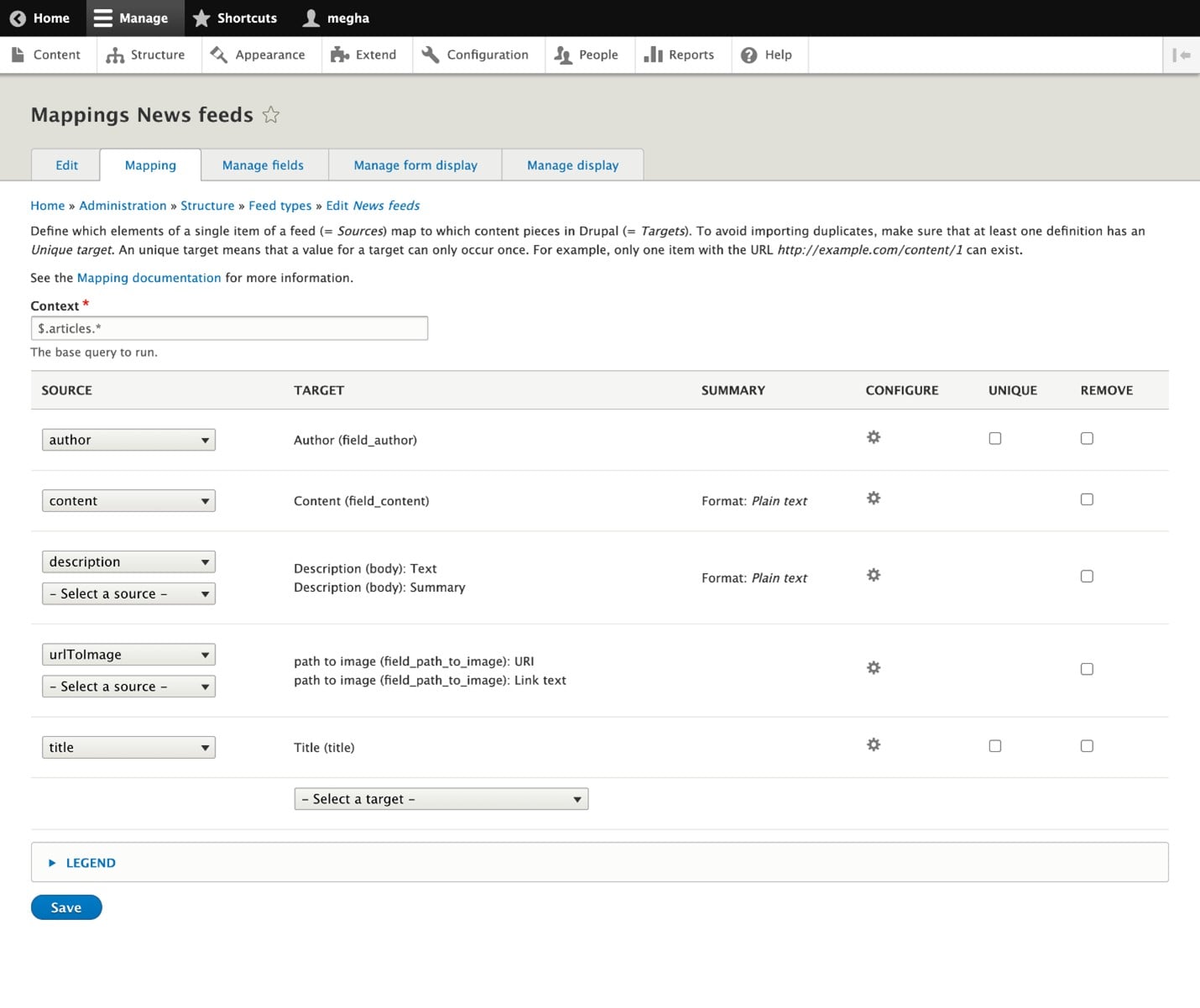**Caption:**

This screenshot showcases an application interface focused on managing news feed mappings in a content management system. 

**Top Navigation Bar:**
- **Title:** "Home" with a back arrow for navigation.
- **Section:** "Manage."
- **Right Side Buttons:**
  - Shortcut button with a star icon.
  - Profile picture named "Mega."

**Primary Menu:**
Beneath the navigation bar, there is a menu with the options: 
- Content
- Structure
- Appearance
- Extend
- Configuration
- People
- Reports
- Help

**Page Title:**
- "Mapping News Feeds" with a star icon.

**Section Tabs:** 
- Edit Mapping
- Manage Fields
- Manage Form Display
- Manage Display
- (Currently active) Mapping

**Breadcrumb Navigation:**
- Home > Administration > Structure > Feed Types > Edit News Feeds

**Description:**
A detailed explanation of how to map elements from a feed source to targets in Drupal, emphasizing the need for unique target definitions to avoid duplicates. An example URL is provided with a link to "mapping documentation" for more information.

**Content Input Area:**
- **Context Field:** Allows input with a description indicating "the base query to run."

**Mapping Table:**
The table contains multiple rows with dropdown menus for mapping various fields:
1. **Author Row:**
   - Target: Author
   - Other columns (Summary, Configure, Unique, Remove): Empty
2. **Content Row:**
   - Target: Content
   - Summary: Format (Plain Text)
   - Other columns (Unique, Remove, Configure): Empty
3. **Description Row:**
   - Target: Description, Body, Text
   - Summary: Format (Plain Text)
   - Other columns (Unique, Remove, Configure): Empty
4. **URL Row:**
   - Source: Path to Image Field
   - Target: Image URI
   - Other columns (Unique, Remove, Configure): Empty
5. **Title Row:**
   - Target: Title
   - Other columns (Summary, Configure, Unique, Remove): Empty

**Additional Dropdowns:**
- **Selected Target:** Nothing selected
- **Legend:** Nothing selected

**Action Button:**
- A blue "Save" button at the bottom of the screen to apply the mappings.